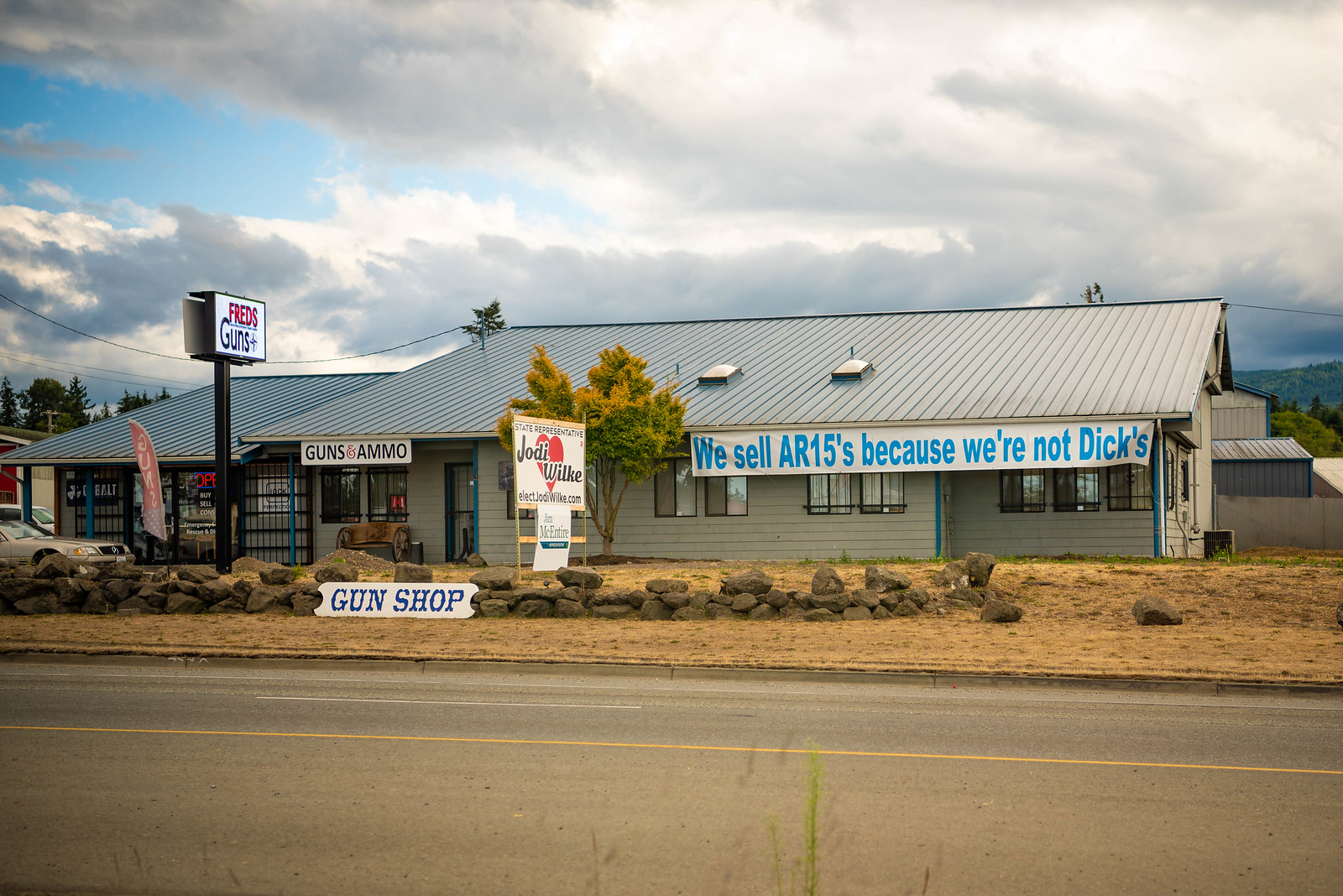This photograph captures the exterior of a quaint, one-story gun shop that resembles a small house. The structure features a steep, sloped roof that appears to be made of metal, colored in shades of silver and gray. At the front of the building, a modest, white sign with blue Old West-style lettering identifies the establishment as a "Gun Shop." Adding to the visual narrative, a large white banner stretches across the façade, boldly declaring in blue text, "We sell AR-15s, because we're not dicks." 

To the left of the building, a gold-colored sedan is parked, providing a sense of scale and setting. The backdrop of the scene includes a dynamic sky, a mixture of blue expanse partially obscured by dramatic, dark storm clouds interspersed with patches of white, adding a contrasting element to the overall composition.